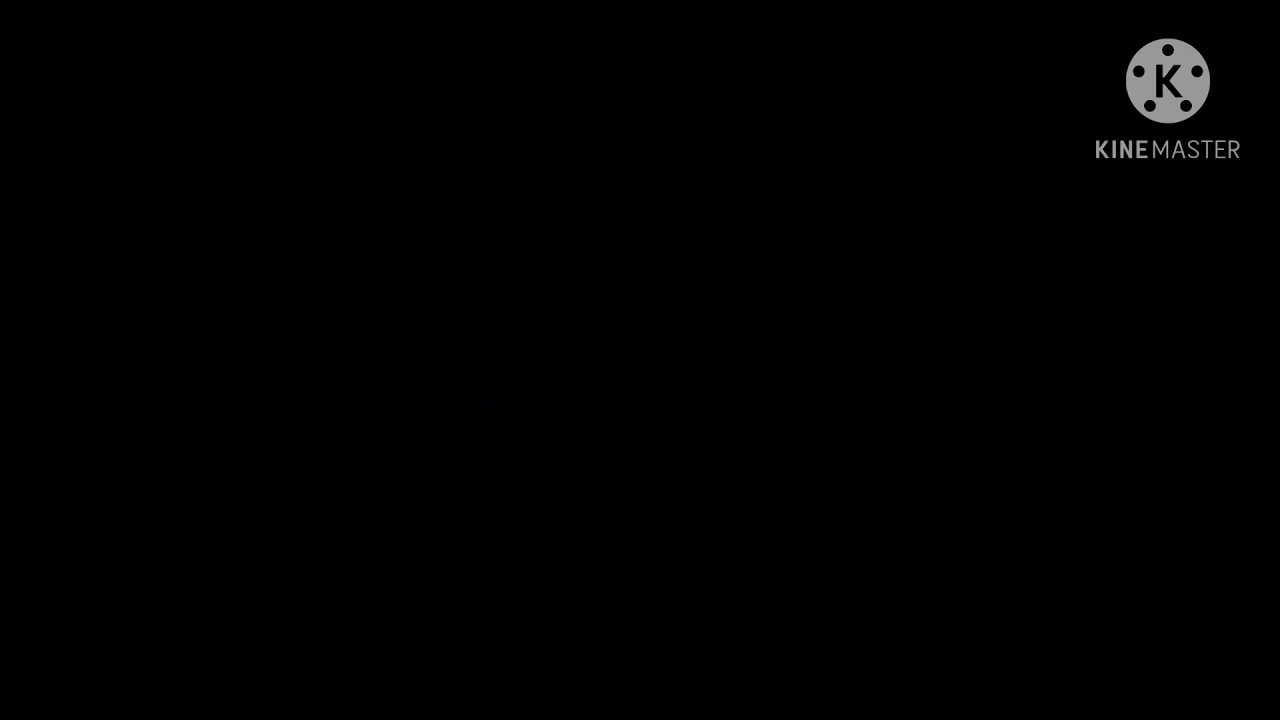The image is completely black, with the only detail being a logo in the top right-hand corner. The logo consists of a gray circle with a capital letter "K" in the center. Inside the circle, there are five black dots positioned at roughly 12 o'clock, 3 o'clock, 5 o'clock, 7 o'clock, and 9 o'clock, resembling spokes on a wheel or holes in a reel tape. Below the circle, the text "KINEMASTER" is displayed, with "KINE" in a bold, medium-gray font and "MASTER" in a lighter, thinner gray font. The overall design of the circle gives the impression of a gear or hubcap, suggesting a potential automotive association.